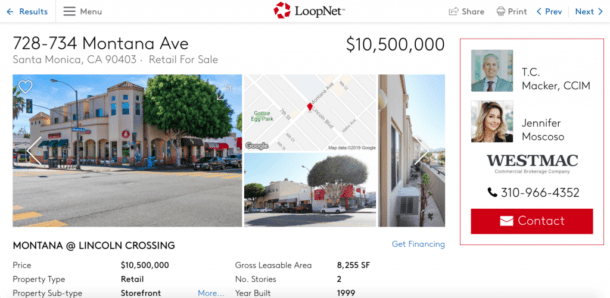This is a detailed descriptive caption for an image showing a screenshot of a website:

---

The screenshot captures the top portion of a website with a clean, white background. In the upper-left corner, there is a blue font text reading "Results," accompanied by a blue left-pointing arrow. Adjacent to this, towards the right, are three horizontal gray lines labeled "Menu." Centered at the top is a circular icon featuring red arrows pointing clockwise, with the text "LoopNet" in black font beside it. To the right of this central section are "Share" and "Print" buttons.

Beneath this banner, there is a search result entry. It prominently features the address "728-734 Montana Avenue" at the top, with the text "Santa Monica, CA 90403. Retail for sale" in gray font below it. To the right of the address, a price tag of "$10,500,000" is displayed. 

Below this information, the screenshot includes a large image of the listed property—a substantial store situated on a corner with a large tree in front. To the right of this image is an embedded Google Map view, pinpointing the property's location. Further down, another image shows a more distant perspective of the same building.

---

The caption offers a thorough and structured description of the screenshot, covering every pertinent detail.